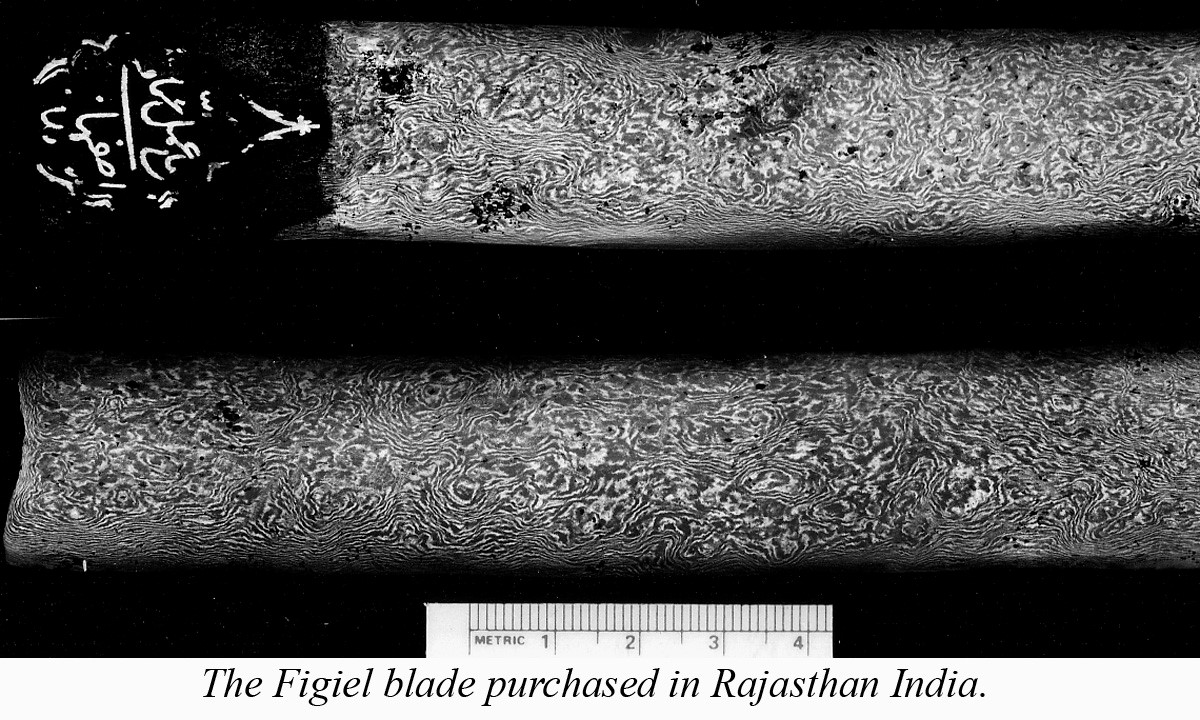This indoor black-and-white photograph features two intricately designed sword blades horizontally positioned against a black background. The top blade is adorned with swirling patterns and what appears to be Arabic or Urdu script, while a blurb points towards this writing. The bottom blade spans the entire width of the image, from left to right. A metric ruler marked with centimeter measurements (1, 2, 3, 4) lies beneath the blades, offering a sense of scale. The caption at the bottom of the image, in italics, reads: "The Figiel blade purchased in Rajasthan, India."